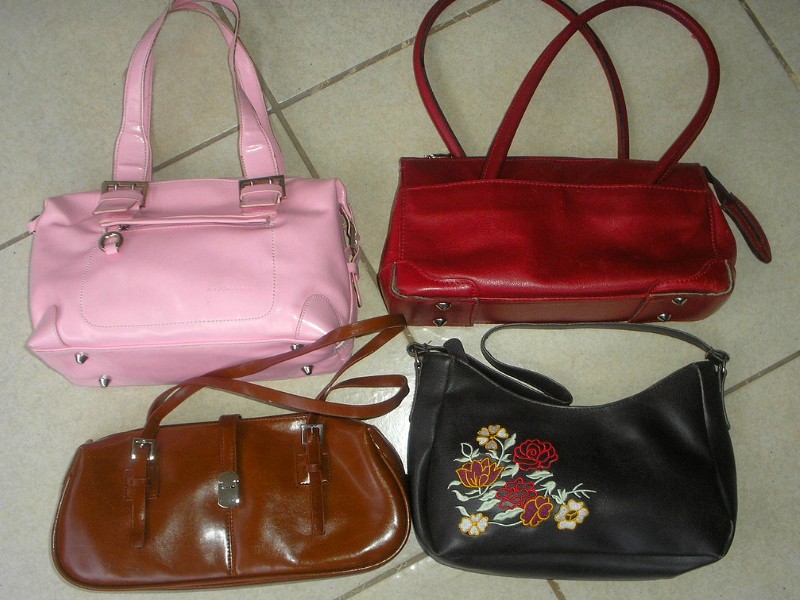This image depicts four handbags arranged on a white tile floor with large tiles outlined in a brown border. Each handbag features a long strap. Starting from the top left, there is a completely pink handbag with two thick handles and four metal balls on the bottom. Adjacent to it, in the top right, is a maroon handbag, also equipped with four metal balls and slender, stiff handles. In the bottom left corner, a brown handbag showcases a single silver buckle, featuring non-stiff, skinny handles. The final handbag, situated in the bottom right corner, is predominantly black with a striking floral pattern on its left-hand side. This pattern consists of red and white flowers, some with hints of yellow. The black handbag has a single non-stiff handle, accentuating its intricate design of red roses, yellow flowers, and distinctive white leaves.